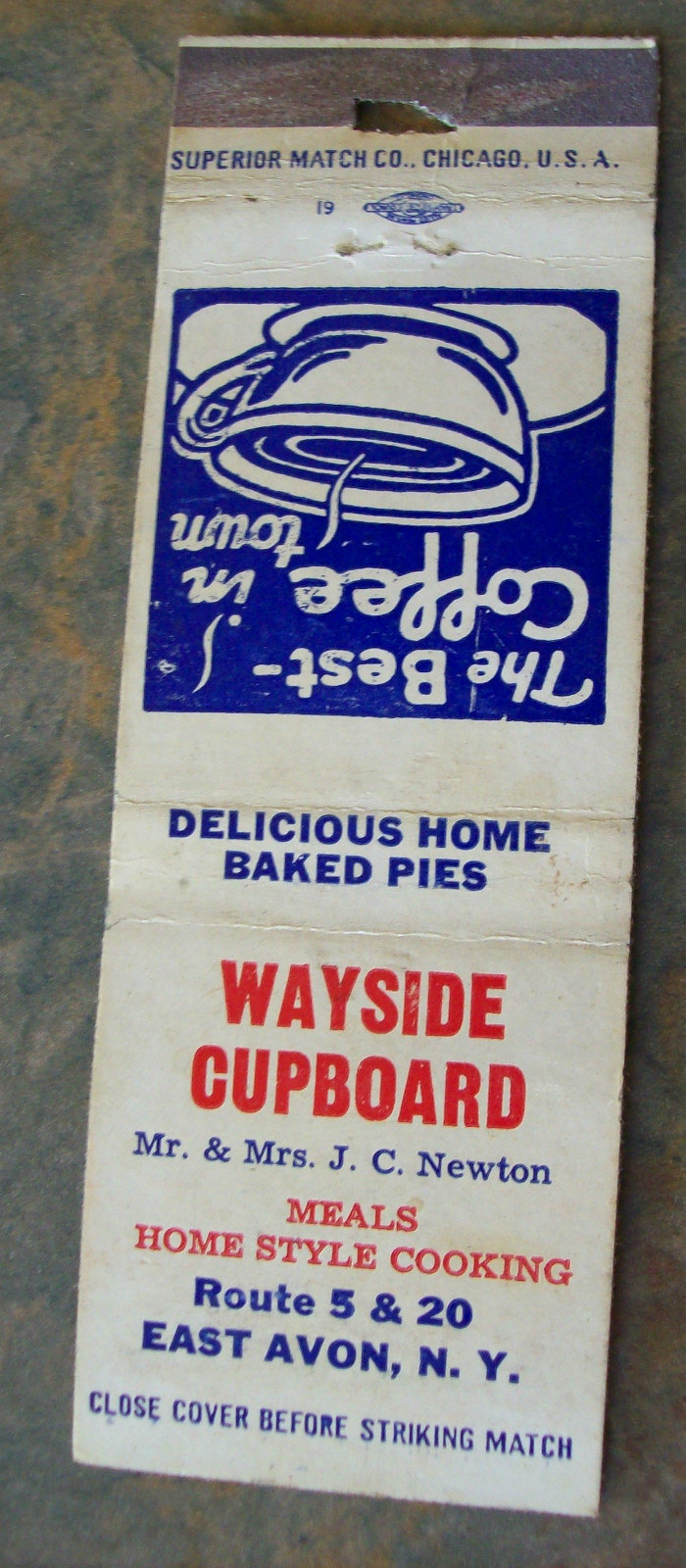This rectangular image captures a worn, vintage matchbook laying facedown, revealing both the front and back covers. The matchbook, showing clear signs of use with a well-worn striking strip and a hole marking its center, prominently features the text "Superior Match Company, Chicago, USA" beneath the strip. 

On what would be the front cover, there's a detailed illustration of a steaming coffee cup paired with the slogan "The Best Coffee in Town" in blue and white. The middle section, bridging the front and back covers, showcases the inviting phrase "Delicious Home-Baked Pies." Further down, the matchbook's front advertises "Wayside Cupboard" in red, followed by "Mr. and Mrs. J.C. Newton" in blue, and "Meals, Homestyle Cooking" also in red. The address "Route 5 and 20, East Avon, New York," along with a safety reminder to "Close Cover Before Striking Match," is presented in blue text. The entire matchbook is set against a white background, enhanced by its red and blue print and imagery.